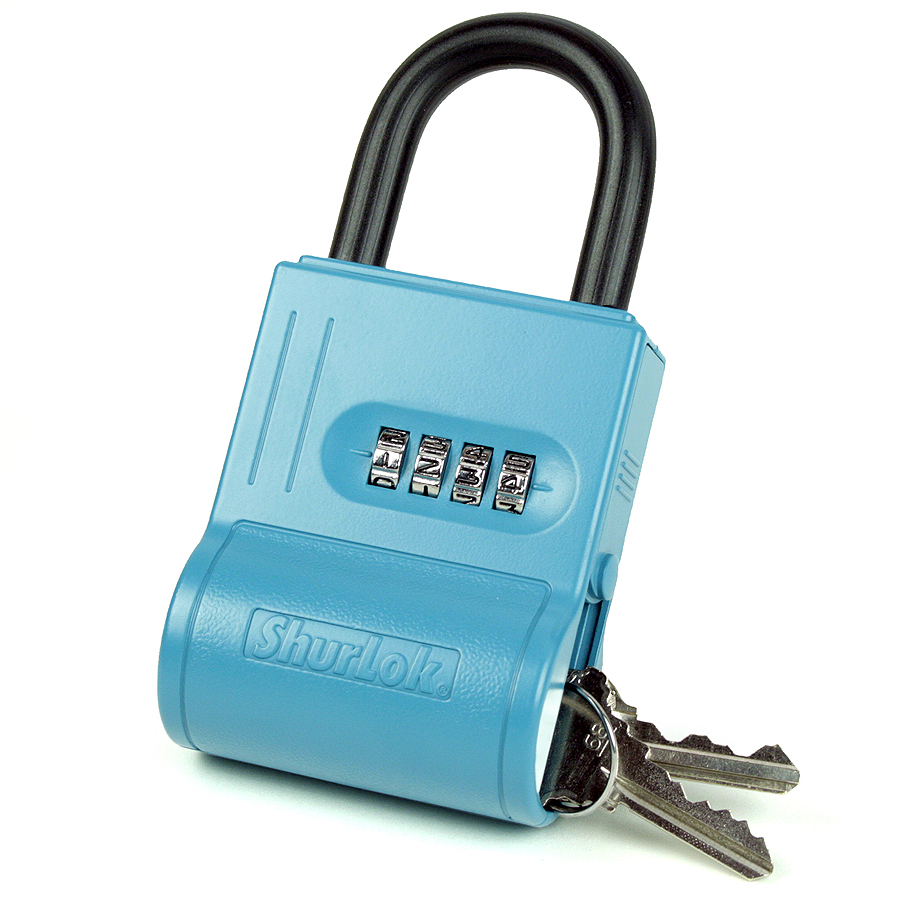This image showcases a distinctive padlock branded "SHURLOK" (with the "S" and "L" capitalized) designed for securing items like lockers or bikes. The lock's body is light blue, possibly plastic or metal, and features a unique compartment for storing items. This compartment currently holds two brass house keys partly protruding from a small inset. The combination dial, composed of four silver number wheels, is prominently displayed, currently set to "1234." The top part of the lock, the shackle, is black and forms a closed loop, ensuring the lock is engaged. The whole setup is against a plain white background.